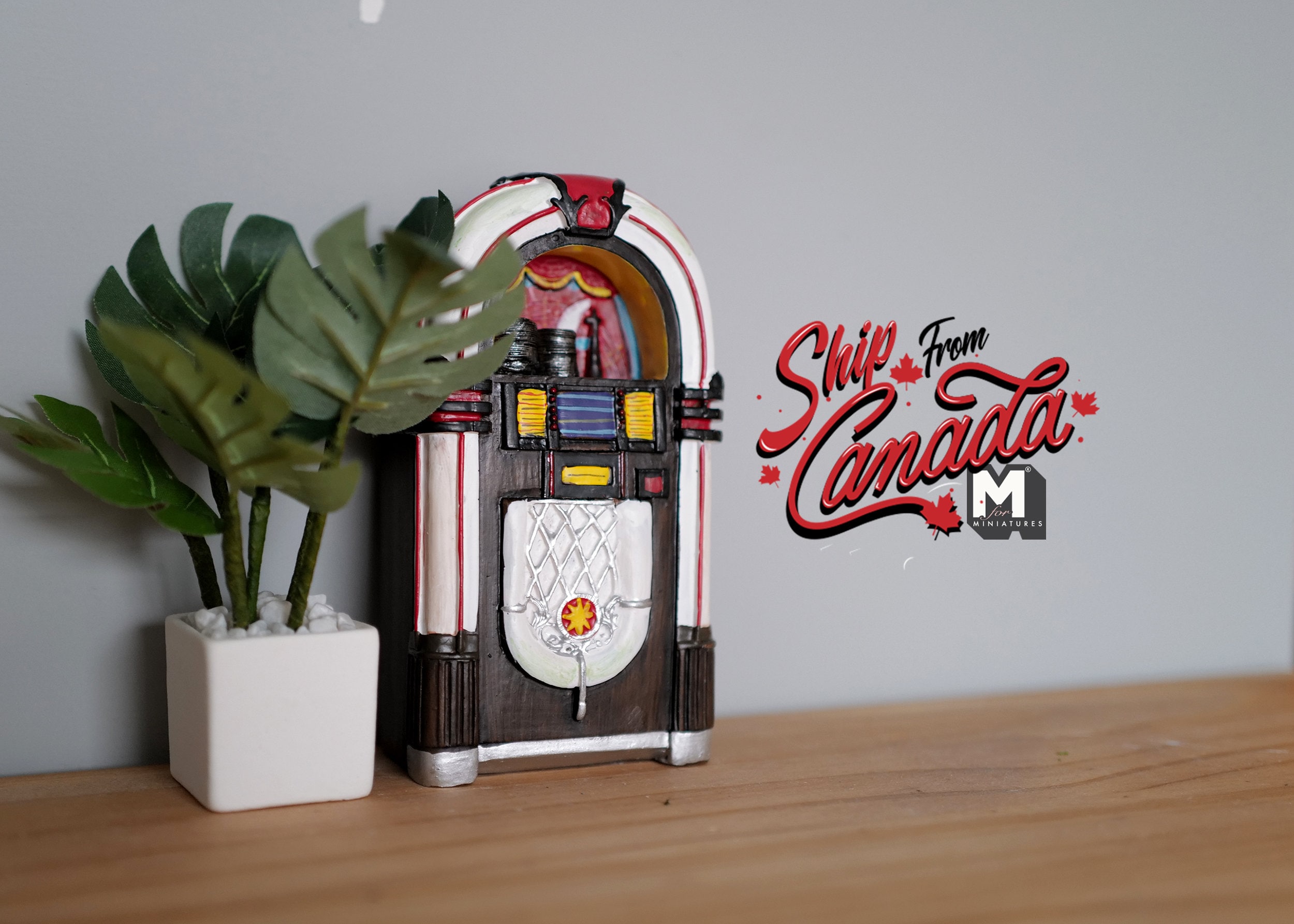This is a detailed color photograph featuring a meticulously crafted model jukebox and a model planter, both placed on a light brown wooden desk. The background wall is a light gray, creating a neutral backdrop that highlights the models. The jukebox is a classic retro style with a wooden exterior, accented by a white border at the curved top, which has a red line running through it. The jukebox's selection buttons are painted a bright orange. To the left of the jukebox, there is a square white planter filled with stones and a large leafy green plant, emphasizing the detailed craftsmanship of the miniatures.

On the right side of the image, digitally inserted text in an elaborate style reads "ship from Canada" with the words "ship" and "Canada" in red cursive, and "from" in black. Scattered around the text are small red Canadian maple leaves, adding a decorative touch. Below this, there is a white and gray logo with a large "M" at the top, followed by the number "4" in cursive, and the word "miniatures" in regular text beneath it. This composition suggests that the image is a promotional photograph for a miniature company named M4 Miniatures.